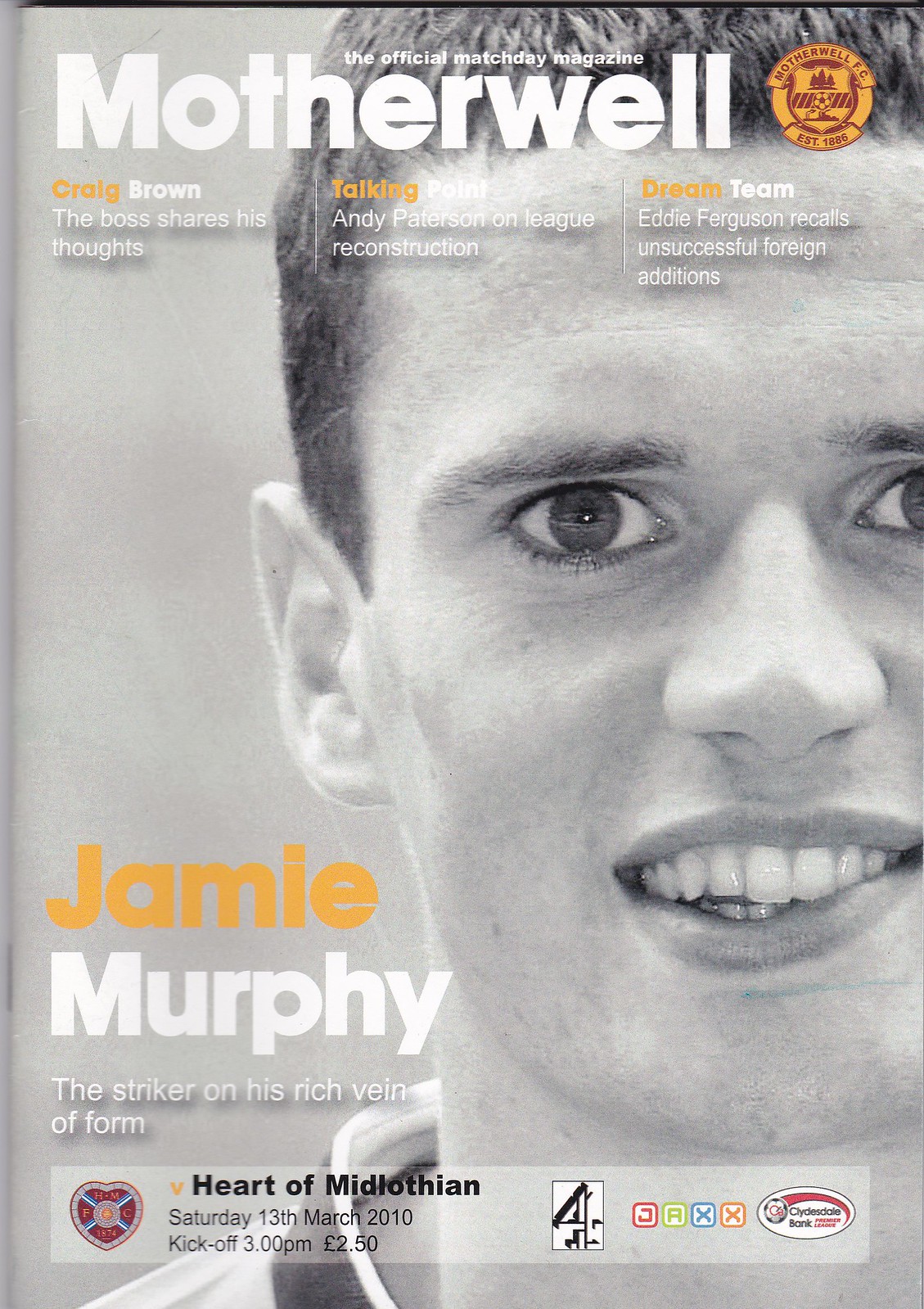The magazine cover is a close-up, black-and-white photograph focusing on a young man's face, where you can distinctly see his eyes, nose, mouth, one ear, and short hair. Dominating the top portion of the cover is the large white title "MOTHERWELL" alongside a red and yellow logo that reads "MOTHERWELL FC" with small text noting "the official Match Day magazine." Below this, large bold text announces "JAMIE" in yellow and "MURPHY" in white, identifying the featured individual. Beneath his name, the text elaborates with "The striker on his rich vein of form." The bottom section of the cover includes a gray banner with black text specifying the details of the match: "Heart of Midlothian, Saturday, 13th March 2010, kickoff 3pm." Additionally, smaller text sections highlight other features: "Craig Brown, The Boss Shares His Thoughts," "Talking Point, Andy Patterson on Legal Reconstruction," and "Dream Team, Eddie Ferguson Recalls Unsuccessful Foreign Additions."